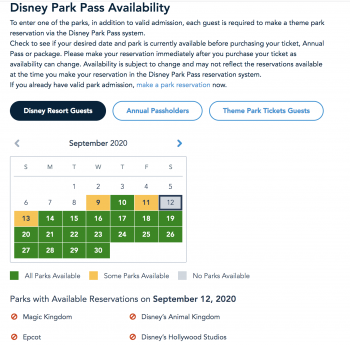The image depicts a website interface for checking Disney Park Pass availability. At the top, the header is printed in a dark blue or black font and reads "Disney Park Pass Availability." Following this, the page provides details about the pass system.

Below the header, a darkly colored background tab labeled "Disney Resort Guests" is displayed in white text. Adjacent to it are two tabs, both with a white background and light-to-medium blue outlines. One tab reads "Annual Pass Holders," combining the words “Pass Holders” into a single term with capitalized initials (AP). The other tab says "Theme Park Ticket Guest," with each word's first letter capitalized.

Further down, the interface shows navigation arrows on either side—left and right—to scroll through the calendar. In the center, the text "September 2020" is prominently displayed, accompanied by a calendar layout with the days of the week denoted as S, M, T, W, T, F, S.

The calendar highlights the following dates:
- Days 1 through 8: White background
- Day 9: Yellow background
- Day 10: Green background
- Day 11: Yellow background
- Day 12: Gray background with a blue-purple border
- Day 13: Yellow background
- Days 14 through 30: Green background

The background colors indicate levels of park availability: green for all parks available, yellow for some parks available, and gray for no parks available.

At the bottom of the calendar, a note specifies the park availability for September 12th, 2020:
- Magic Kingdom
- Epcot
- Disney's Animal Kingdom
- Disney's Hollywood Studios